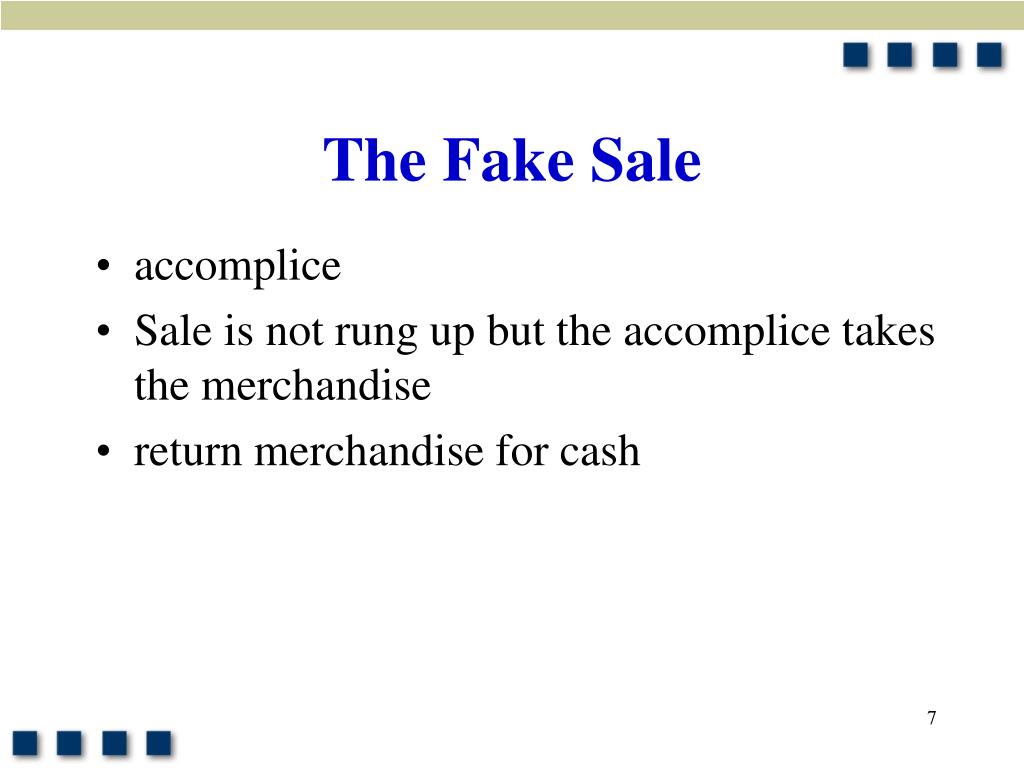This horizontal rectangular image, resembling a PowerPoint slide, features a light gray or beige horizontal stripe at the top. Below this stripe, on the far right, is a vertical lineup of four dark blue squares, mirrored at the bottom left corner of the image, framing the slide against its white background. Dominating the center of the slide, in large blue letters, is the title "The Fake Sale," with each word capitalized. Directly beneath the title, three bullet points in black text detail a retail scam: "Accomplice," "Sale is not rung up, but the accomplice takes the merchandise," and "Return merchandise for cash." This appears to serve as an advisory notice, likely aimed at retail workers to highlight common fraudulent activities.